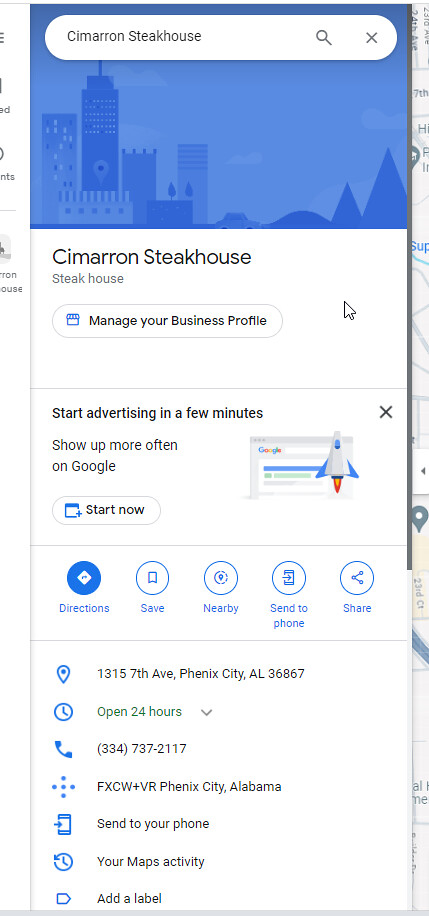This image is a detailed screenshot of Google Map search results for "Samaritan's Steakhouse." At the top, the search query is clearly visible, confirming that the user was looking up this specific establishment. Below the search bar, the name "Samaritan's Steakhouse" appears prominently, along with a link labeled "Manage this business," suggesting that the viewer might be the business owner or someone with administrative privileges, likely intending to update information or review feedback.

The screenshot showcases various typical Google Map functionalities. A prompt box encourages users to "Start advertising in a few minutes," indicating options for business promotion. Icon buttons for "Directions," "Save," "Nearby," "Send to phone," and "Share" are visible, offering standard navigational and sharing tools. The steakhouse's address is listed, pinpointing its location in Phenix City, Alabama, and it is noted as "open 24 hours," providing convenience for potential visitors. The phone number is also displayed for direct contact.

Additionally, the screen includes references to "FXCW, Phenix City, Alabama" and options for "Send to your phone," "Your map activity," and "Add a label," which are typical features for personalized map management and ease of use. The overall design is encapsulated within a long rectangular layout, dominated by whites and blues, which are characteristic of Google's clean and user-friendly interface.